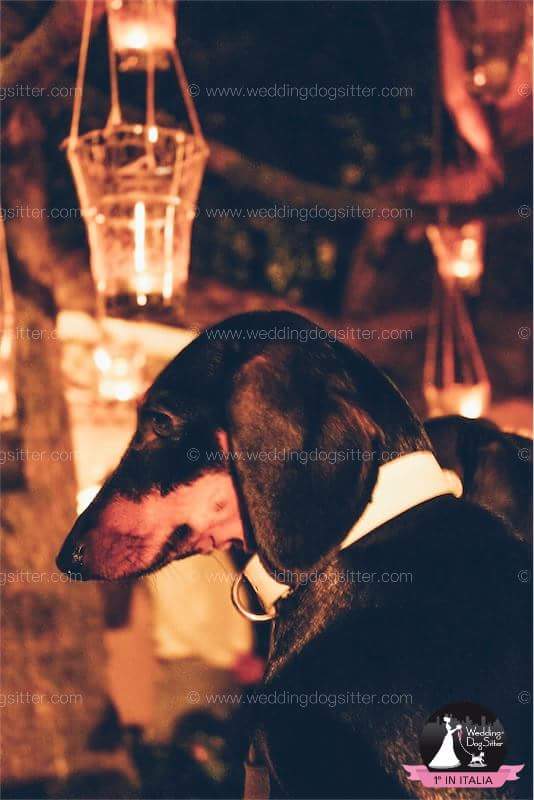The promotional image for a wedding dog sitter service prominently displays a basset hound sitting and looking to the left. The dog's top half is mostly a glossy black coat, with its mouth and cheeks area illuminated to a light brown, possibly due to sunlight. The dog wears a white collar. The background features a warm, elegant setup akin to a wedding, complete with hanging lanterns or candle holders. The grassy ground is visible with some lines or sticks scattered on it. The watermark, comprising the copyright symbol "©" and the website "www.weddingdogsitter.com," repeats across the image.

In the bottom right corner, there's a logo showing a bride walking a small dog on a leash, facing right, accompanied by the text "Wedding Dog Sitter" and "F in Italia," indicating the service's prominence in Italy. The overall ambiance of the photograph is warm and well-lit, suggesting it was taken at night. The combination of details underscores the professional and elegant nature of the wedding dog sitter service being promoted.